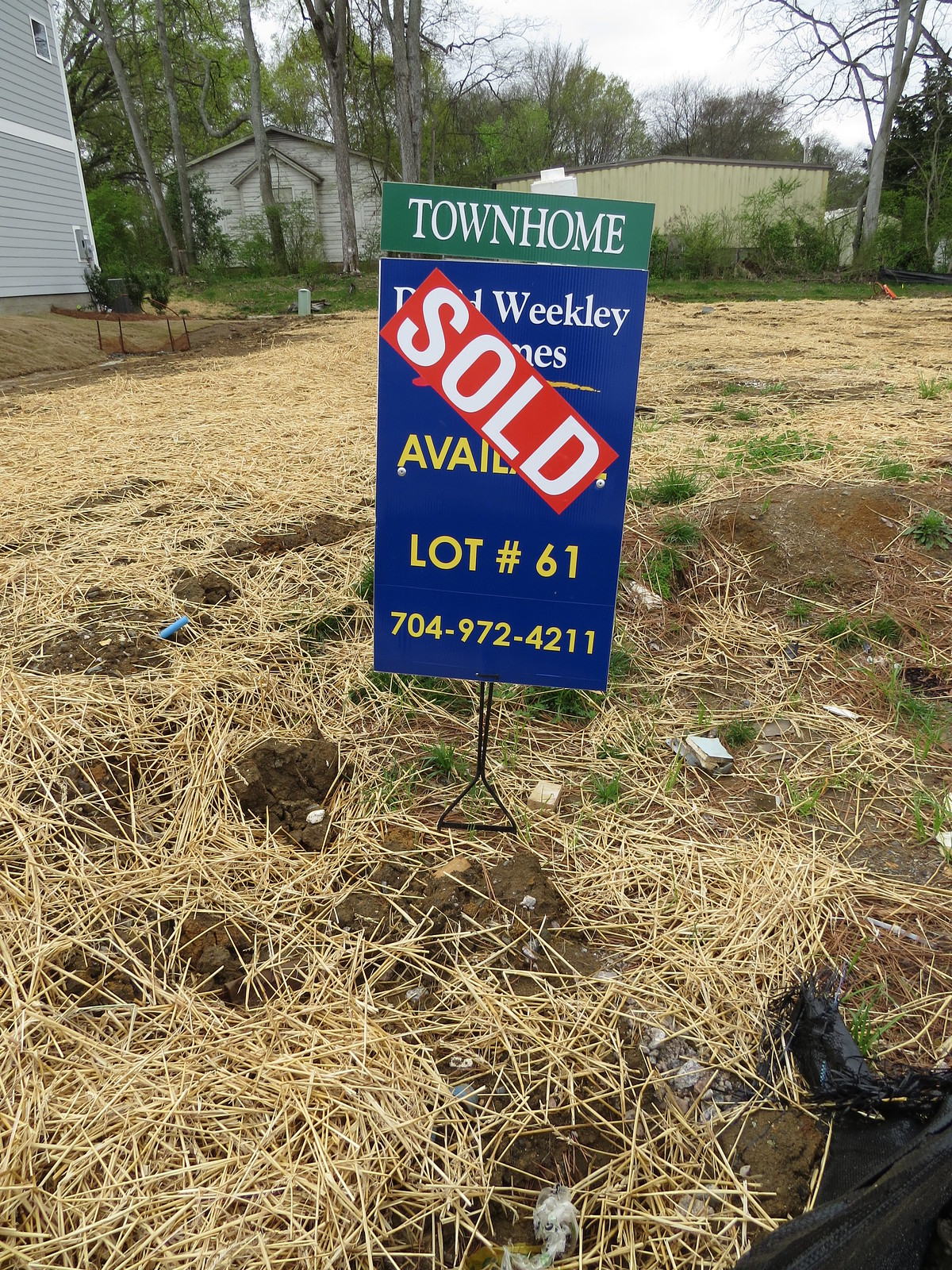The image captures a portrait view of an empty lot nestled between two houses. At the top of the image, there's a partial view of buildings and tall trees against a gray sky. Occupying about 80% of the frame, the background ground consists of weeds, dirt, hay, and patches of grass, contributing to a rough, undeveloped look. 

At the center focal point of the photo stands a sign on a black, ground-anchored post. The top section of the sign is green with white text that reads "Townhome." Below, the main part of the sign is blue with white and yellow text, which is mostly obscured by a prominent red diagonal sticker with white text stating "SOLD." Partial text visible includes words like "weekly" and a contact number "61 704 972 4211," indicating that the lot was available for sale before being sold.

To the left of the lot, there is a house with gray siding, and in the background are two sheds—one gray and one yellow. The lower right foreground displays a black tarp on the ground amidst the patches of dirt, hay, and clumps of grass. This thorough portrayal emphasizes that the once available large lot, now sold, offers substantial space, possibly for building a significant structure.